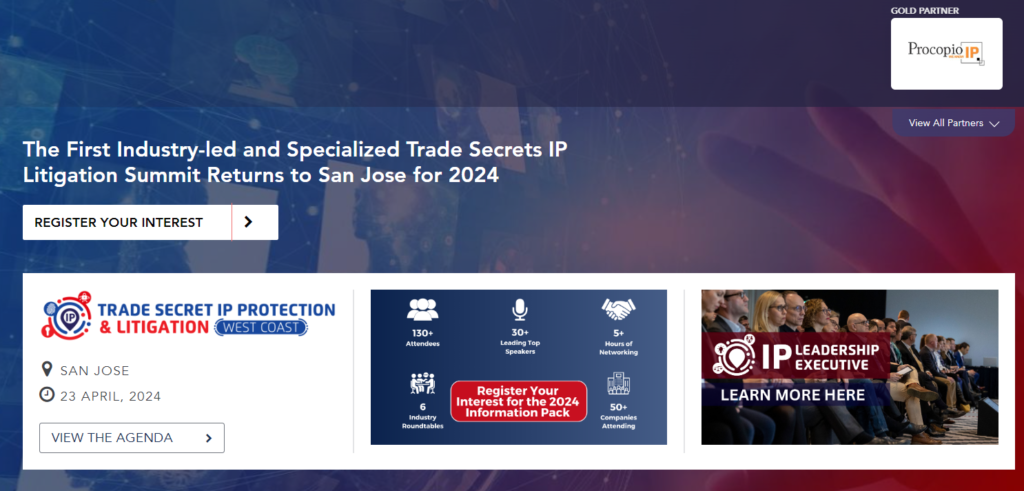The image depicts a section of a webpage showcasing details about the 2024 Trade Secret IP Protection and Litigation Summit in San Jose. Starting from the lower right corner, there is a photograph of an audience seated in an auditorium with a red banner labeled "IP Leadership Executive." Underneath this image, there's a "Learn More Here" link.

To the left, another section highlights event statistics with icons above each text: 
- "130+ attendees"
- "30+ leading top speakers"
- "5+ hours of networking"
- "50+ companies attending"
- "6 industry round tables"

Below these statistics, a prominent red button invites users to "Register Your Interest for the 2024 Information Pack."

Leftward still, the page presents key event details with icons:
- "Trade Secret IP Protection and Litigation West Coast"
- Location: San Jose
- Date: 23 April 2024
- A clickable "View the Agenda" button

Above this section, another button, "Register Your Interest," stands out.

Further up, text announces, "The first industry-led and specialized Trade Secrets IP Litigation Summit returns to San Jose for 2024."

In the upper right corner, an area titled "ProCipico IP" is marked as "Gold Partners," with an adjacent "View All Partners" button.

The webpage's visual theme is primarily white, featuring a background image of a hand, enhancing the professional and clean layout.